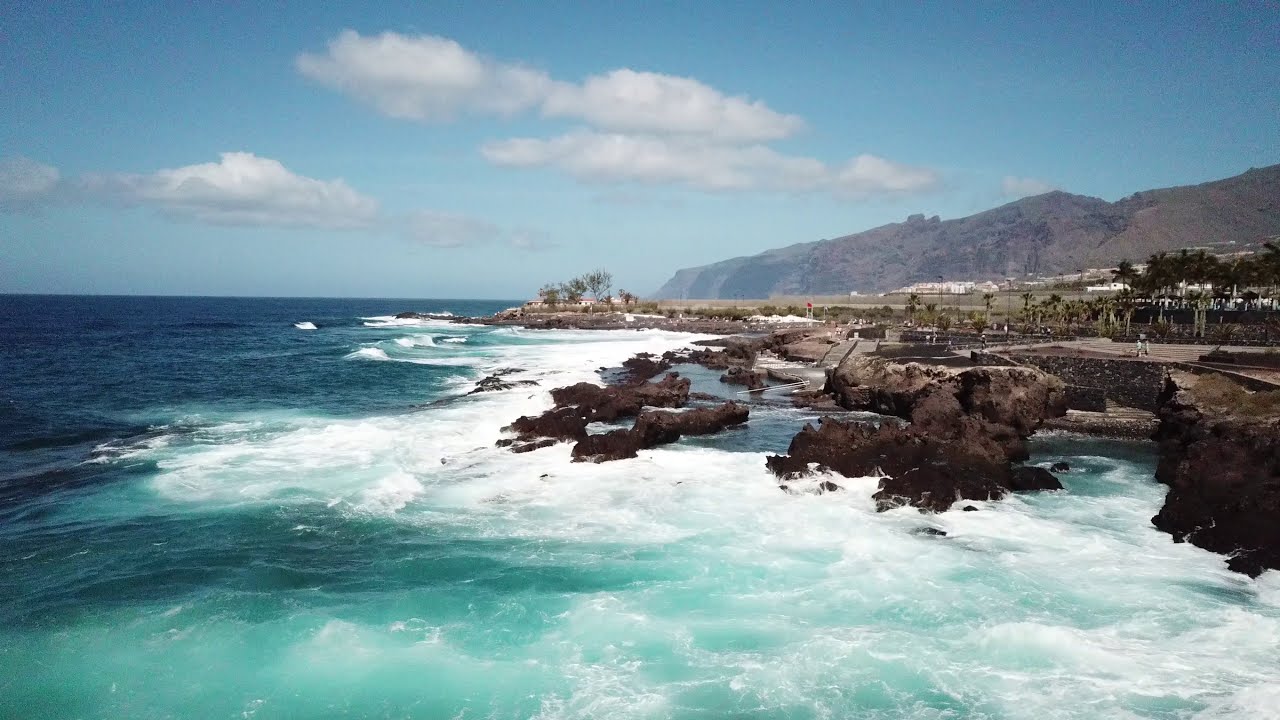The image captures a breathtaking coastal scene from an elevated vantage point, possibly taken from a drone or a high edifice. Below, the wild, turquoise ocean waves crash vigorously against a rocky coastline, creating striking contrasts of white foam against the deep blue water. The coastline itself is composed of dark volcanic rocks that transition to lighter brown hues as they extend inland. A series of stone walkways and a rock pool, framed by a white barrier, lend an intriguing man-made touch to the natural beauty.

To the right, the land features sporadic vegetation, including some palm trees, interspersed amid dry, rocky terrain. In the mid-ground, a small concrete area is visible, along with a person in white walking casually in the distance. Further inland, a small village of white buildings nestles among the trees and rocks.

In the background, a towering mountain range dramatically rises from the sea, culminating in steep cliffs that dominate the horizon. The sky above is mostly clear with a few puffy white clouds, suggesting a clear, sunny day. This serene yet dynamic setting encapsulates the raw beauty and power of nature, highlighting the dramatic interaction between land and sea.